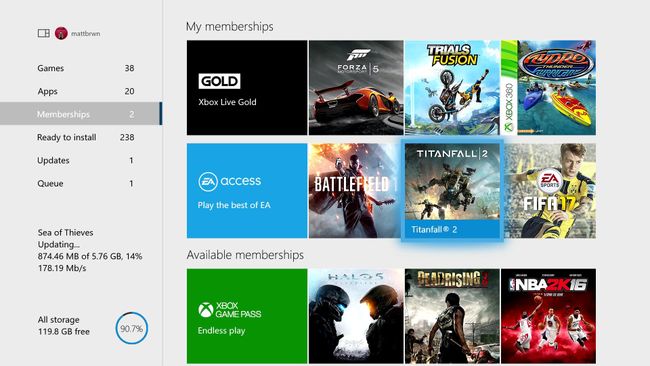**Detailed Caption:**

The image displays a membership overview page of an account named Matt Breen. Dominating the top left corner is Matt Breen’s profile picture encased in a circle. To the right of the profile picture, "Matt Breen" is clearly displayed. Beneath the name, various statistics are listed: Games (38), Apps (20), Memberships (2), Ready to Install (238), Updates (1), and Queue (1).

A segment of the page indicates the game "Sea of Thieves" is currently updating. The storage information reveals 119.8 GB of free space, with a progress circle showing 90.7% completion of an unspecified task. 

Adjacent to the "Memberships" section, there is a blue scroll bar against a grey background.

On the right side of the interface, under the heading "Mine Memberships," there are three rows and four columns showing different memberships and games. 

The first row lists:
1. Gold: Xbox Live Gold
2. Forza 5
3. Trios Fusion
4. Nydro

The second row shows:
1. Access: Play the Best of EA
2. Battlefield

This detailed layout provides a clear and organized view of Matt Breen’s gaming and membership details on the platform.